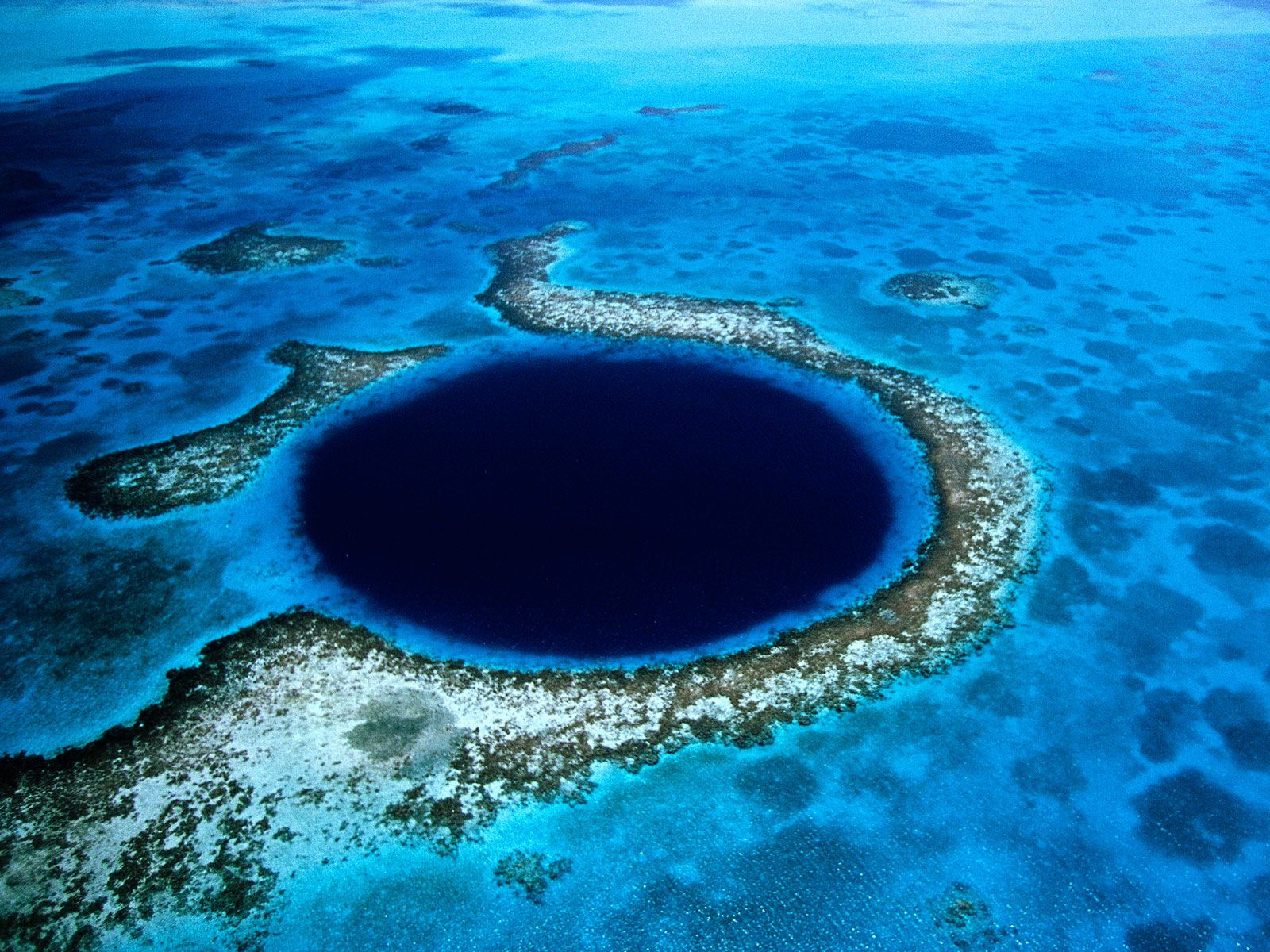This detailed aerial photograph captures the Samaesan Hole in Thailand, a striking underwater feature in an incredibly vibrant blue ocean. Dominating the image is the Samaesan Hole, a massive, nearly perfect circular trench in the earth, marked by its very dark, almost black center, indicative of its significant depth. Surrounding this abyss is a shallower, vividly blue stretch of water, where the sea bed is visible, showcasing patches of sandy bottom interspersed with dark areas likely representing algae or rocky formations. The periphery of the hole is encircled by a rocky, reef-like structure that forms an island-like shape, filled with terrain varying in greens, beiges, and dark rocks. The water clarity outside the central abyss offers a stark contrast, as it appears much lighter in blue and incredibly clear, further highlighting the dramatic depth of the Samaesan Hole. The image, slightly landscape-oriented, features a cloud-speckled sky, enhancing the natural beauty of this striking marine landscape.